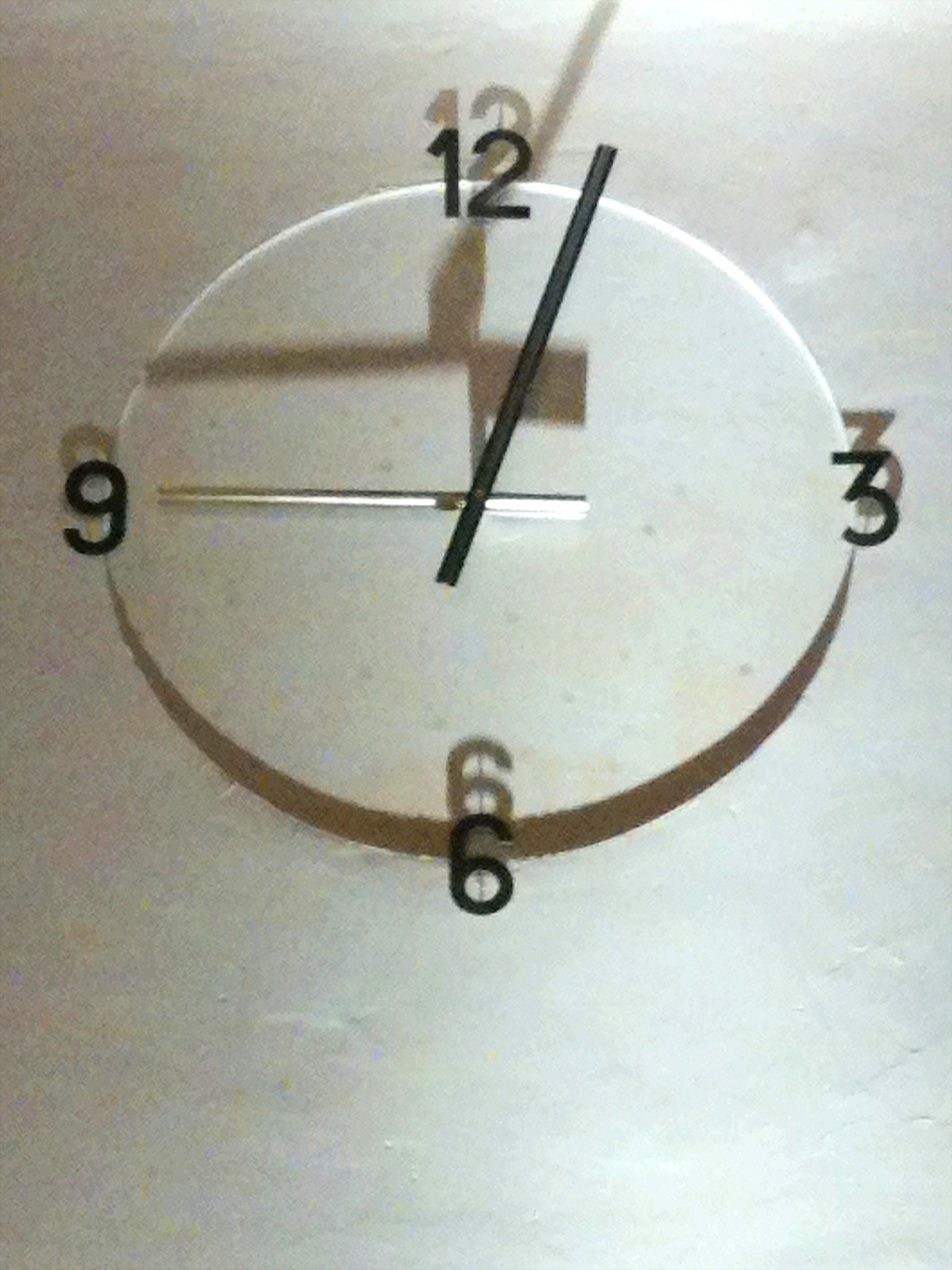This is a photograph of a highly minimalist analog clock set against a white concrete wall. The clock has no discernible frame, giving it a seamless appearance as if the clock face is an indent into the wall itself. The clock features only four black numbers: 12 at the top, 3 on the right, 6 at the bottom, and 9 on the left. The hour hand, which is slightly shorter and metallic, points directly at the number 9, while the long black minute hand hovers between the 12 and the 1, indicating a time of approximately 9:01. The image resolution is somewhat low, with noticeable graininess, possibly accentuating the sleek and stark design of the clock, which lacks any extra markings or embellishments.